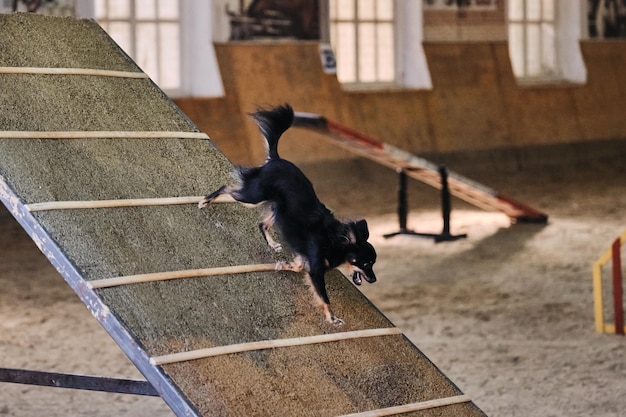This detailed photo captures a small, black and tan long-haired Chihuahua running eagerly down a segmented wooden ramp with stops that prevent it from sliding. The dog, with its mouth open and tail up, moves energetically to the right, displaying an almost perfect form with one paw forward and the others extended behind. The setting appears to be an expansive indoor arena with a sand or sawdust floor, which is ideal for dog training. Glimpses of a dog agility course surround the energetic Chihuahua, including a seesaw and another ramp in the background secured by a black holder, highlighting the training environment. The arena's walls are partially wooden, topped with three white-painted windows that obscure the outside view, emphasizing the focused interior space dedicated to dog agility and training activities.